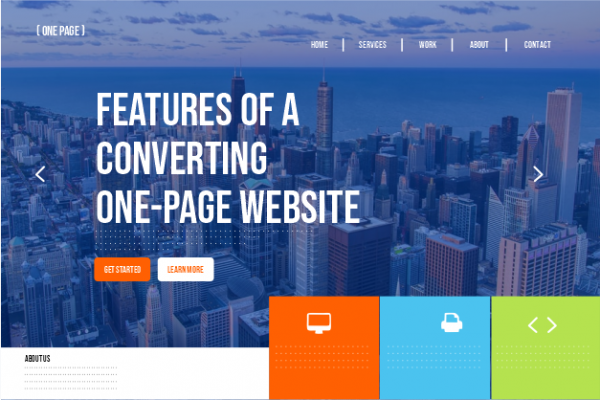The image features a website advertisement for web design services. The layout is landscape-oriented, indicating it's probably viewed on a computer screen. The background showcases a cityscape next to a body of water, suggesting a major waterfront city like San Francisco or an Asian metropolis, all under a blue overlay that enhances the readability of the white text.

In the upper left-hand corner, the logo "OnePage" is displayed. The navigation tabs include Home, Services, Work, About, and Contact. Prominently, there is left-aligned text that reads “Features of a Converting OnePage Website.” Below this text, two buttons prompt user interaction: an orange "Get Started" button and a white "Learn More" button.

Further down, three clickable rectangular boxes in orange, blue, and green are visible. The orange box contains an icon resembling a Macintosh desktop computer, the blue one displays a printer, and the green one has two arrows pointing left and right.

An "About Us" section is partially visible, with text in the bottom left that is too small to read clearly. The overall design indicates that this website is promoting a web design service, focusing specifically on OnePage website designs.